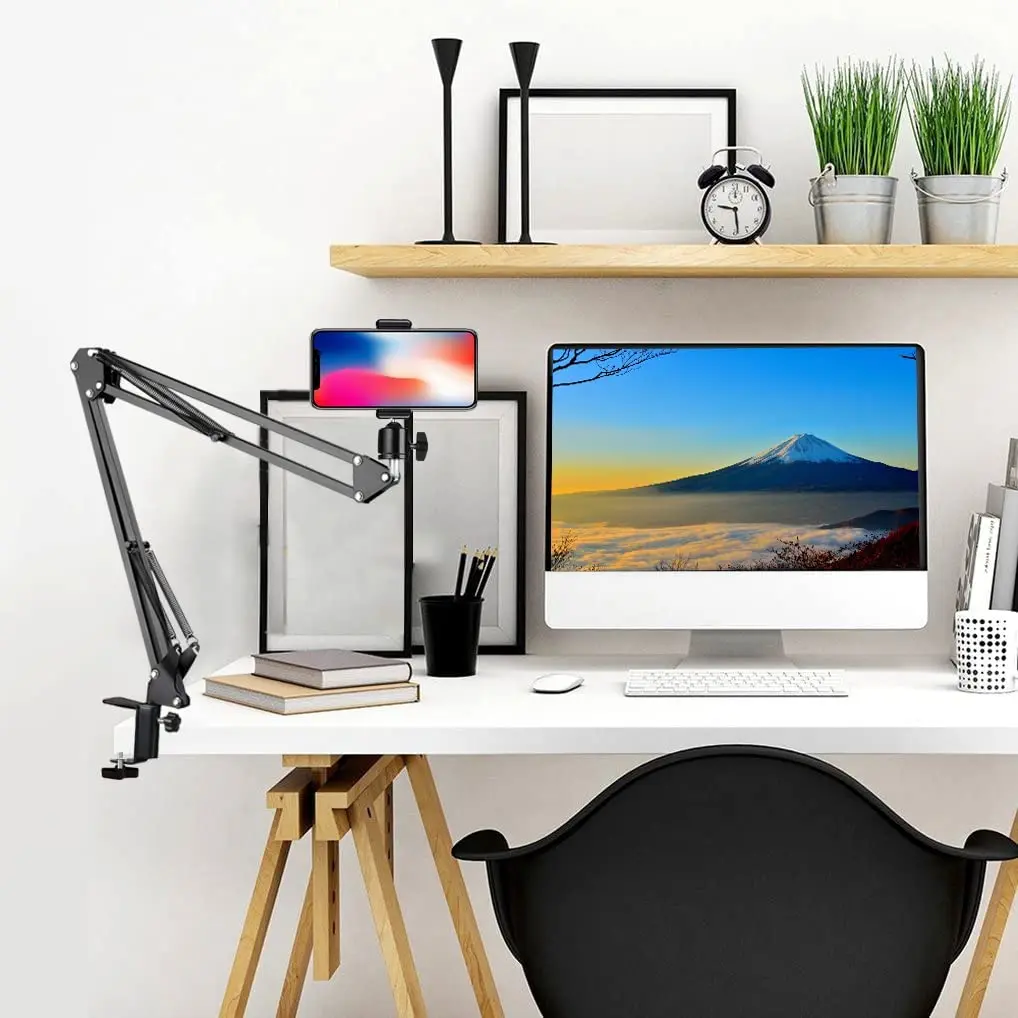The image depicts a meticulously arranged office setup centered around a white desk on wooden sawhorse legs, with a black chair in front of it. On the desk sits a computer monitor displaying a picturesque scene of a fog-covered, sunlit mountain under a blue sky. To the left of the monitor is a stand holding a blurry phone.

Above the desk is a wooden shelf adorned with various items. Dominating the right side of the shelf are two silver pails filled with lush, green ornamental grass. In the middle, a black alarm clock is perched, showing the time as 2:30, though the numbers appear backward. Toward the left end of the shelf are two tall, black candle stands framing a black picture frame whose contents are indiscernible.

On the desk, directly in front of the monitor, is a black glass filled with pencils, along with a computer mouse and keyboard. To the left side, a stack of two books lies beneath the phone stand—the top book with a smaller gray cover, the bottom larger with a tan cover. Additionally, a black and white cup and several gray-covered books are positioned to the right. The arm of the phone holder is visible on the left side of the image. Behind all this, another black frame picture, empty or indistinct, contributes to the elegant yet functional aesthetic of the workspace.